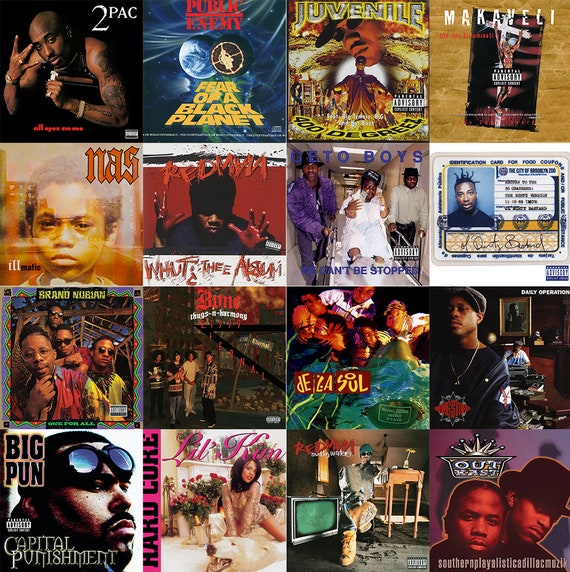This detailed square image is a 4x4 grid collage of 16 hip-hop and rap album covers, each one arranged evenly across four rows. The albums span influential artists primarily from the 1990s. Starting from the upper left, the first row features Tupac Shakur, followed by 'Fear of a Black Planet' by Public Enemy, '400 Degrees' by Juvenile, and an album titled 'Machiavelli.' The second row includes an album by Nas, Redman's 'What Thee Album,' the Ghetto Boys' 'We Can't Be Stopped' with its distinctive spelling "G-E-T-O," and a unique item resembling a food coupon or certification card. The third row begins with Brand Nubian, Bone Thugs N Harmony, a possibly misspelled and less clear album 'Dejasoul,' and Gang Starr's 'Daily Operation.' The bottom row showcases 'Capital Punishment' by Big Pun, Lil' Kim's 'Hardcore,' another Redman album, and finally OutKast's 'Southernplayalisticadillacmuzik,' partially identified with 'Southern Play' visible. Each album cover represents iconic music from the era, with imagery including space themes, a license-like depiction, and parental advisory labels, reflecting the cultural and artistic style of 1990s rap music.